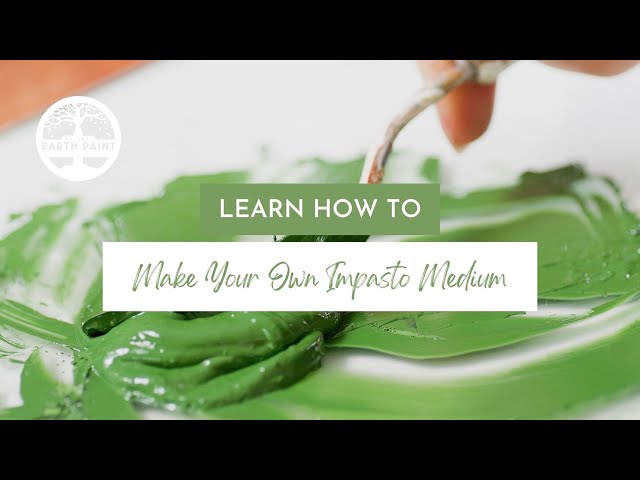This professionally photographed, landscape-oriented cover image illustrates the process of making your own impasto medium. Dominated by an earthy, dark green paint, the image captures an artist’s fingers gripping a metal tool used to manipulate the paint. The action is partially obscured by central text that reads, "Learn how to make your own impasto medium," with "learn how to" in white, all-caps lettering bordered by a green box, and "make your own impasto medium" in cursive within a white rectangular box. In the top-left corner, a white circle logo features the brand Earth Paint, depicting a tree with barren branches rooted in a base of dirt. The image suggests a blend of artistic creativity and hands-on learning, framed by thin black bars above and below the photograph, adding a polished, professional finish to the advertisement.